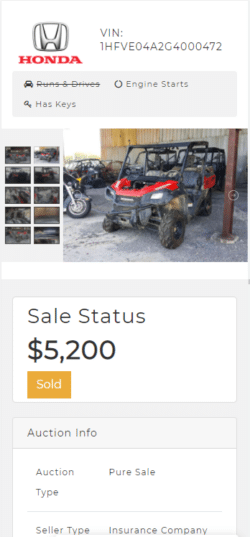A detailed screenshot of a Honda website showcases the brand's distinctive logo positioned at the upper left-hand corner, with the word "Honda" prominently displayed in red letters underneath. Adjacent to the logo, the VIN number 1HFVE04A2G4000472 is clearly visible. Directly below, a gray bar features various vehicle status indicators: an icon of a car labeled "Runs and Drives" is crossed out, while beside it, the phrase "Engine Starts" is displayed. Below the "Runs and Drives" section, a key icon with the label "Has Keys" is present.

Dominating the central portion of the screenshot is an image of the vehicle in question—a robust four-seater, all-terrain vehicle. The ATV is depicted in a striking red color, complemented by a black interior. To the left of this image, a collection of 12 thumbnail photos are arranged vertically, offering viewers an option to click and enlarge for a closer look.

Further information is provided below the main image, stating that the sales status of the vehicle is marked at $5,200. An orange button located beneath this price information indicates that the vehicle has been sold.